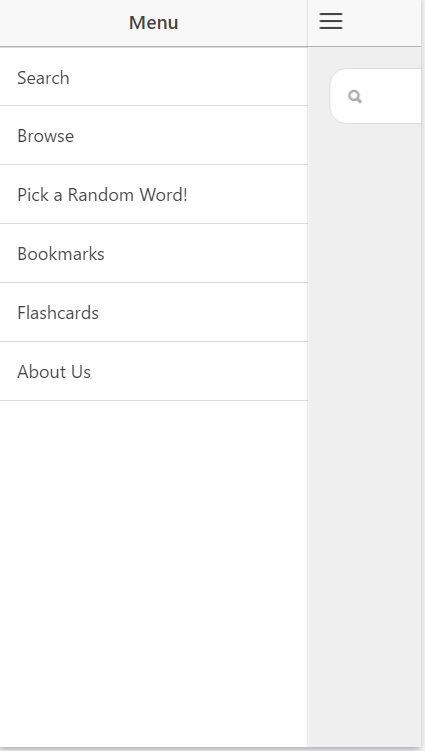The image depicts a website interface with a prominent gray navigation bar at the top labeled "Menu." Within this navigation bar, there is a clickable icon consisting of three horizontal lines, oriented vertically, which likely serves as a menu toggle or hamburger menu.

Directly below the gray navigation bar, a white section contains several navigation options, each listed in light gray text. The first option is labeled "Search," followed by "Browse," and "Pick a Random Word!"—the latter of which notably includes an exclamation point. Further down the list are "Bookmarks," "Flashcards," and "About Us."

On the left side of the white section, situated below the three horizontal lines, is a search icon placed within a white circular bubble. This white section, along with its navigation options, is outlined in light gray on the right side and along the bottom edge. There is no visible outline on the left side or along the top edge of the menu.

The image does not provide a clear context or heading beyond the word "Menu," leaving the specific relation of the flashcards, bookmarks, and other options uncertain.